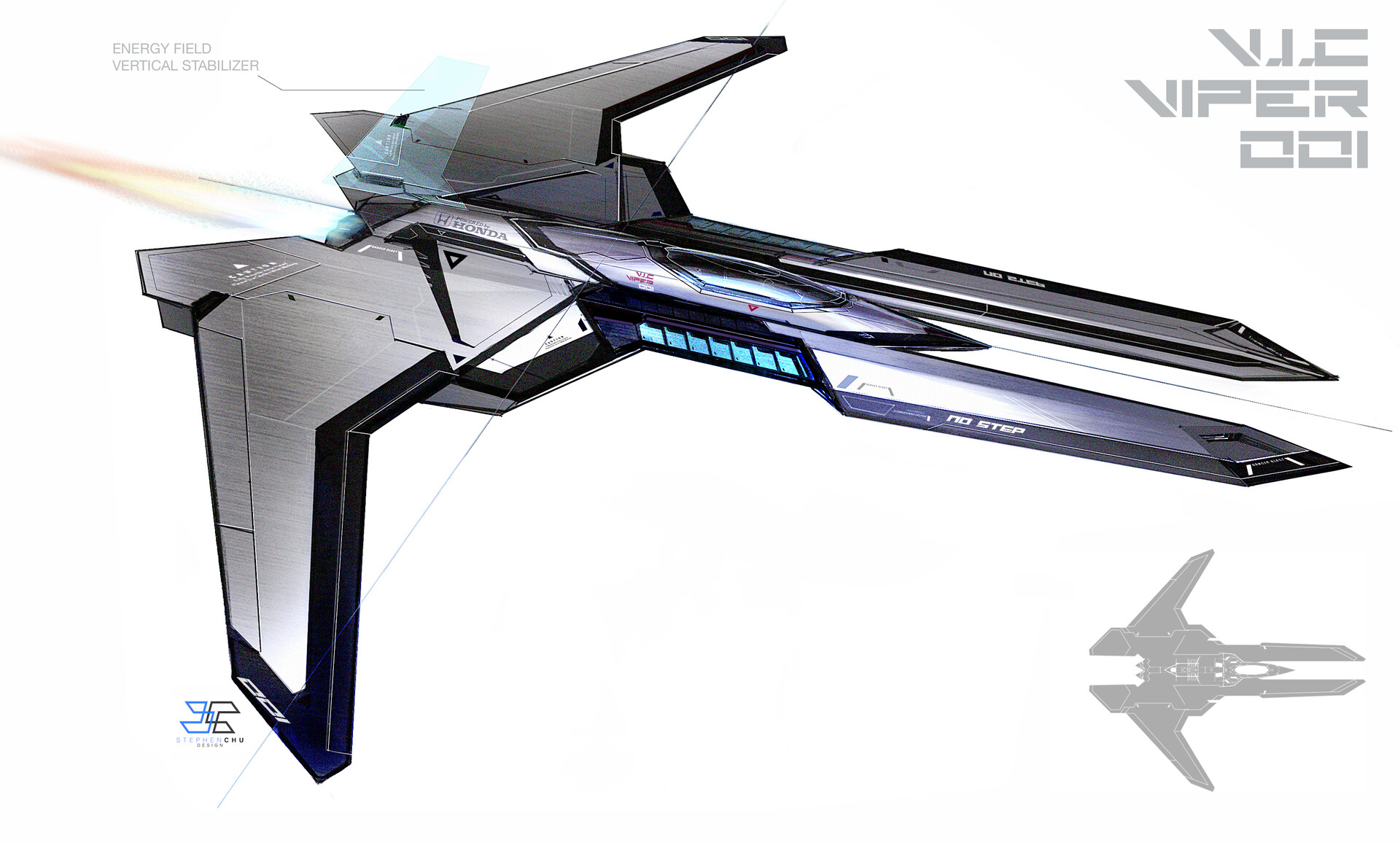The illustration appears to depict a meticulously detailed plane or possibly a model plane, prominently titled "VIC Viper 001" in gray lettering. The top section of the image provides a comprehensive view of the aircraft. The plane itself features a gleaming metallic finish accented with black around the outer edges. Notably, one of the black edges bears the cautionary inscription "no step," a common safety advisory on aircraft. 

The plane is equipped with a jet engine and a pilot compartment labeled "Honda" at the rear. Extending from the pilot compartment are two long passageways with large windows, suggesting these sections are designed for crew members or passengers, potentially indicating the aircraft's suitability for space travel.

The illustration highlights the plane's dual-wing configuration: one wing extends horizontally, while the other extends downward, likely to demonstrate the versatility and configurability of the wings. The detailed rendering and strategic placement of components suggest a highly advanced and functional design, emphasizing both aesthetics and utility.